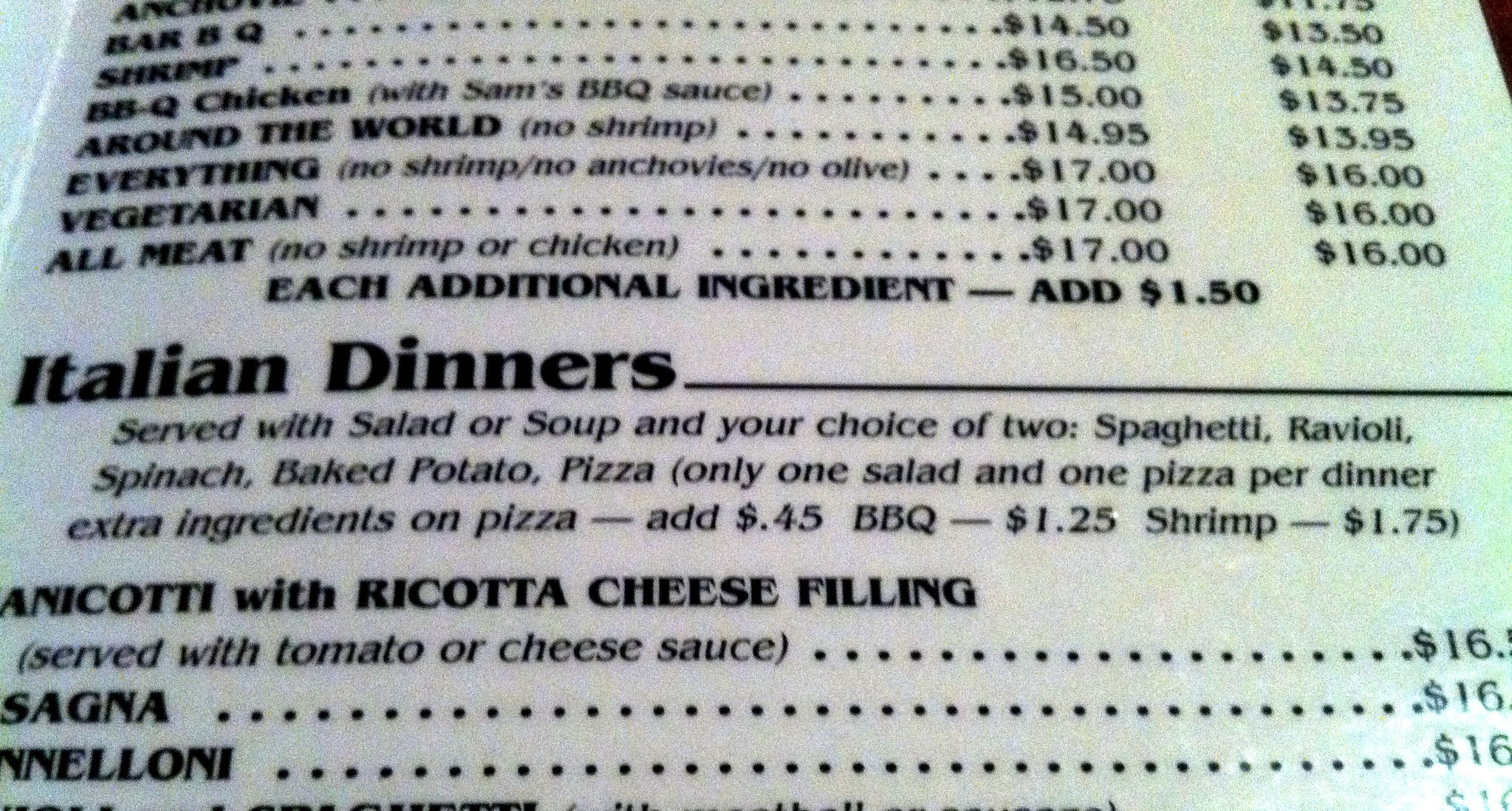The image captures a detailed portion of a restaurant menu, possibly from an Italian eatery. The top section of the menu features various pizza options. Below the pizza listings, there are sections for Barbecue Dinners, something intriguingly labeled as "Everything," and a Vegetarian option.

Further down, the menu details Italian dinners, specifically noting that these meals are served with a choice of salad or soup and two side dishes. The side dish options include spaghetti, ravioli, spinach, baked potato, or pizza, with the stipulation that only one salad and one pizza can be chosen per dinner. Extra ingredients for pizza are priced at $0.45 each, $1.25 extra for barbecue toppings, and $1.75 extra for shrimp toppings.

Highlighted Italian dishes include manicotti filled with ricotta cheese, available with either tomato or cheese sauce, priced at $16. Lasagna is also offered on the menu. The vegetarian meal is listed at $17, with another size option available for $16. The menu indicates that other dishes similarly have two different price points each.